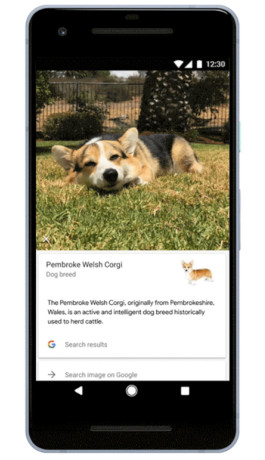In this image, captured from a black smartphone screen, several details are prominent. At the top right corner of the screen, white icons display essential information: the time reads 12:30, alongside icons for the battery, network signal, and Wi-Fi signal. Below these icons, the main focus is an image of a Pembroke Welsh Corgi dog, lying down on a patch of mixed green and brown grass. The Corgi, facing towards the camera, features a coat with black, brown, and white fur.

The background of the dog showcases a fence with dimly lit trees, indicating a distant background, and more brown grass behind the fence. Beneath the dog’s image, white text reads: "Pembroke Welsh Corgi dog breed." To the right of this text, another image of a Corgi, with brown and white fur, is displayed. Accompanying this is an explanatory note: "The Pembroke Welsh Corgi, originating from Pembroke, Wales, is an active and intelligent dog breed historically used to herd cattle."

At the bottom of the screen, the text "Search results" is displayed next to the Google icon, which is colored in red, yellow, green, and blue. The final line reads: "Search image on Google."